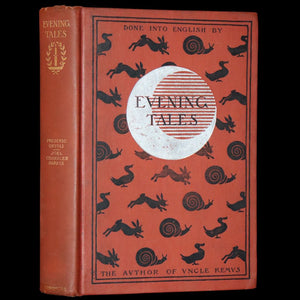This photograph captures a leather-bound book titled "Evening Tales" propped against a black backdrop, which accentuates the book's colors and intricate details. The cover is framed by two black-lined boxes, enclosing the title "Evening Tales" in a prominent font. Below the title, the text "Done into English by the author of Uncle Remy" is barely readable due to its old-fashioned script. The cover and spine feature a collection of animal silhouettes, including a snail, duck, and rabbit, adding a whimsical element to the design. The spine also displays a laurel logo with a candle beneath the title. Central to the cover is a distinctive moon emblem, with a circle and white stripes, contributing to the book's vintage and mystical aesthetic.